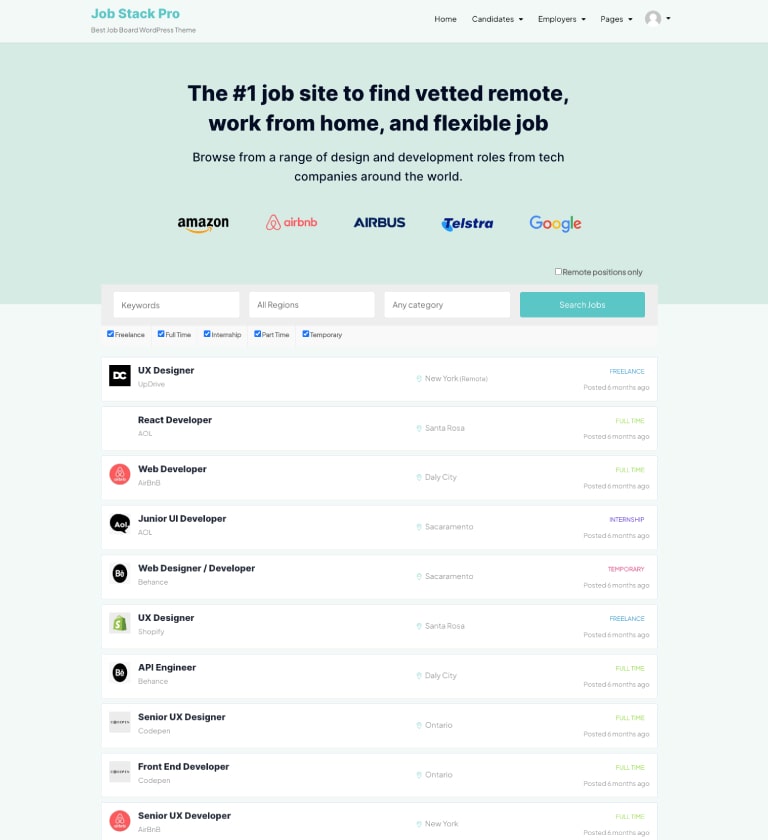This is an image of a website interface with a light gray horizontal bar at the top labeled "Job Stack Pro" in teal on the left side. Beneath this, in smaller text, it reads "Check Jobs WordPress," though the text is too small to clearly decipher. On the right side of the bar, there are several menu options in gray: "Home," followed by "Candidates" with a downward-facing arrow, "Employers" with a similar arrow, "Pages" with another arrow, and a profile button represented by a gray circle with a white silhouette of a person's head and shoulders, accompanied by a downward-facing arrow.

Below this top bar, there is a darker blue or light blue horizontal rectangle. Within this rectangle, towards the middle-left of the page, the text states, "The #1 job site to find vetted remote, work-from-home, and flexible jobs" in bold black letters. Beneath this, in black letters, it reads, "Browse from a range of design and development roles from tech companies around the world."

Further down, logos of several companies are displayed: Amazon with its iconic yellow smile arrow, Airbnb in red, Airbus in bold dark blue letters, Telstra in bold blue letters, and the Google logo with multi-colored letters.

Proceeding further, there are three search boxes: "Keyword" on the middle-left, "All Regions" in the middle, and "Any Category" towards the right, followed by a blue "Search Jobs" button. Above these search bars, there is an empty checkbox labeled "Remote positions only" in black text.

The main content section below this search area lists various job postings. Each posting includes a job title on the left and a location to the right, some of which are too small to read. The listings include:

1. UX Designer
2. React Developer
3. Web Developer (notable for a small rectangular image in a red circle beside it).
4. Junior UI Developer (preceded by a black rectangle with white letters reading "AOL").
5. Web Designer/Developer (accompanied by a black button with white letters "BUB").
6. UX Designer (with a gray horizontal rectangle containing a green suitcase and a white dollar sign).
7. API Engineer (next to a blurred black oval with white letters).
8. Senior UX Designer (beside a nondescript gray rectangle).
9. Front-End Developer (accompanied by another gray rectangle with small, indiscernible text).
10. Senior UX Developer (beside a red circle with a white triangle inside).

The detailed design elements and functional components are geared towards facilitating an efficient job search for users seeking remote, work-from-home, or flexible job opportunities in design and development roles from tech companies globally.